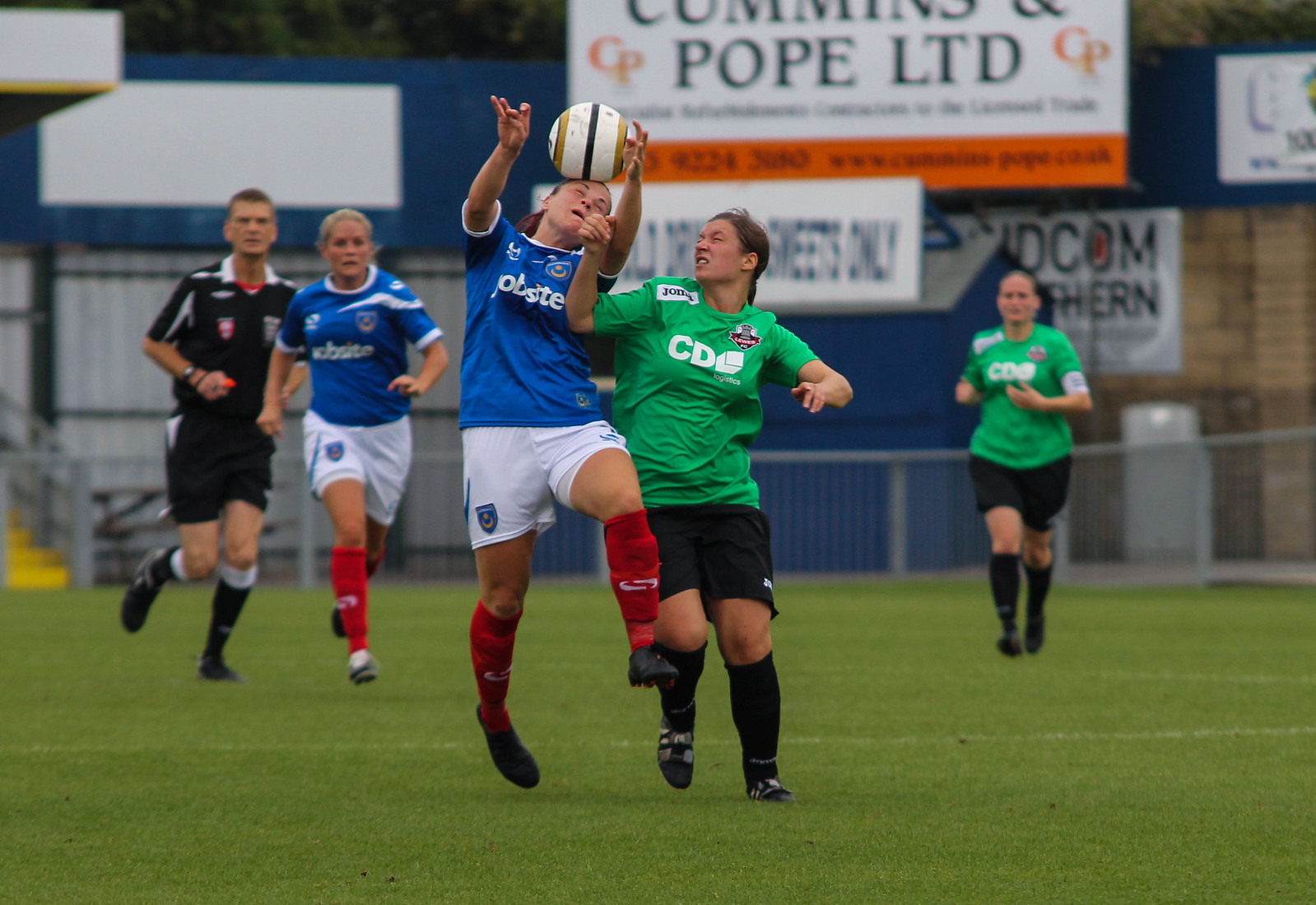The photograph captures an outdoor soccer match on a green, grassy field, likely on an overcast day. Centered in the image are five players in different uniforms: two players in blue jerseys with white shorts, two in green jerseys with black shorts, and one in all black who appears to be the referee. In the midst of action, the player in a blue jersey is visibly jumping up to head the ball, while another player in a green jersey tries to block her. Surrounding them, two other players, one in blue and one in green, are actively participating in the play. In the background, a fence, a blue wall, and a sign with the text "Pope Ltd" can be seen.